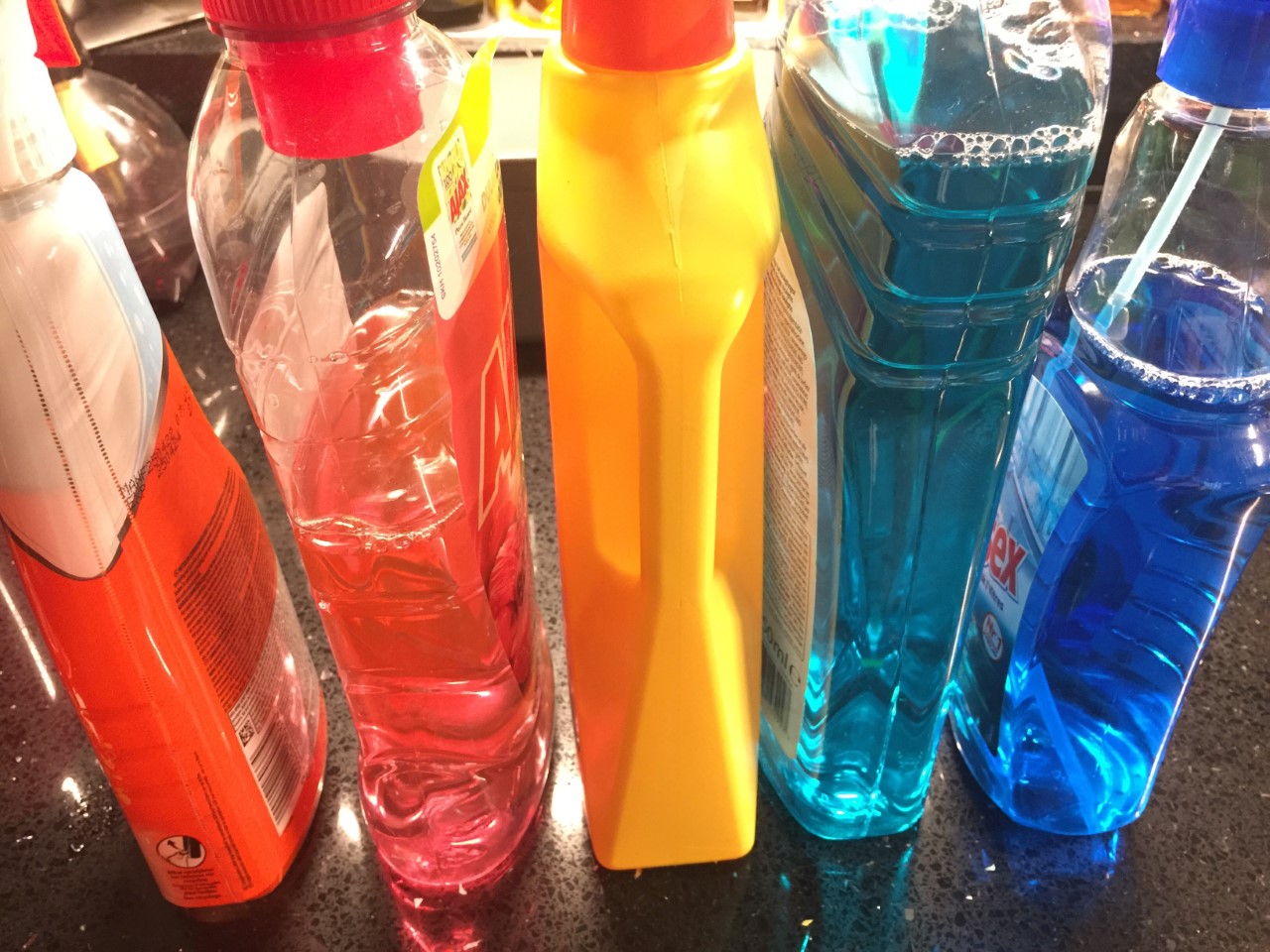This is a close-up, color photograph of five plastic bottles placed on a textured brown surface, likely stone or wood. The shot appears to be taken with a wide-angle lens, capturing the bottles in detail but cropping out the tops and part of the sides.

1. **Leftmost Bottle**: The first bottle on the left is orange at the bottom and white at the top, capped with white. A clear bottle with a red cap and possibly a yellow straw is slightly visible behind it.

2. **Second Bottle**: It is clear and contains a tangerine-colored liquid, about half full, with a red top and a yellow label. The bottle appears slightly crumpled.

3. **Middle Bottle**: This is an opaque yellow plastic bottle, featuring a handle facing the camera and capped with red.

4. **Fourth Bottle**: This clear bottle has a bright sky-blue liquid, nearly full, with horizontal ridges on the top portion. It has a blue cork and possibly a straw inside. 

5. **Rightmost Bottle**: The final bottle is clear with a translucent blue liquid, around two-thirds full, featuring a blue cork and a label that partially reads "Windex."

Reflective elements are visible on the surface, and the far background is not in view, focusing all attention on the bottles which appear to be cleaning supplies.